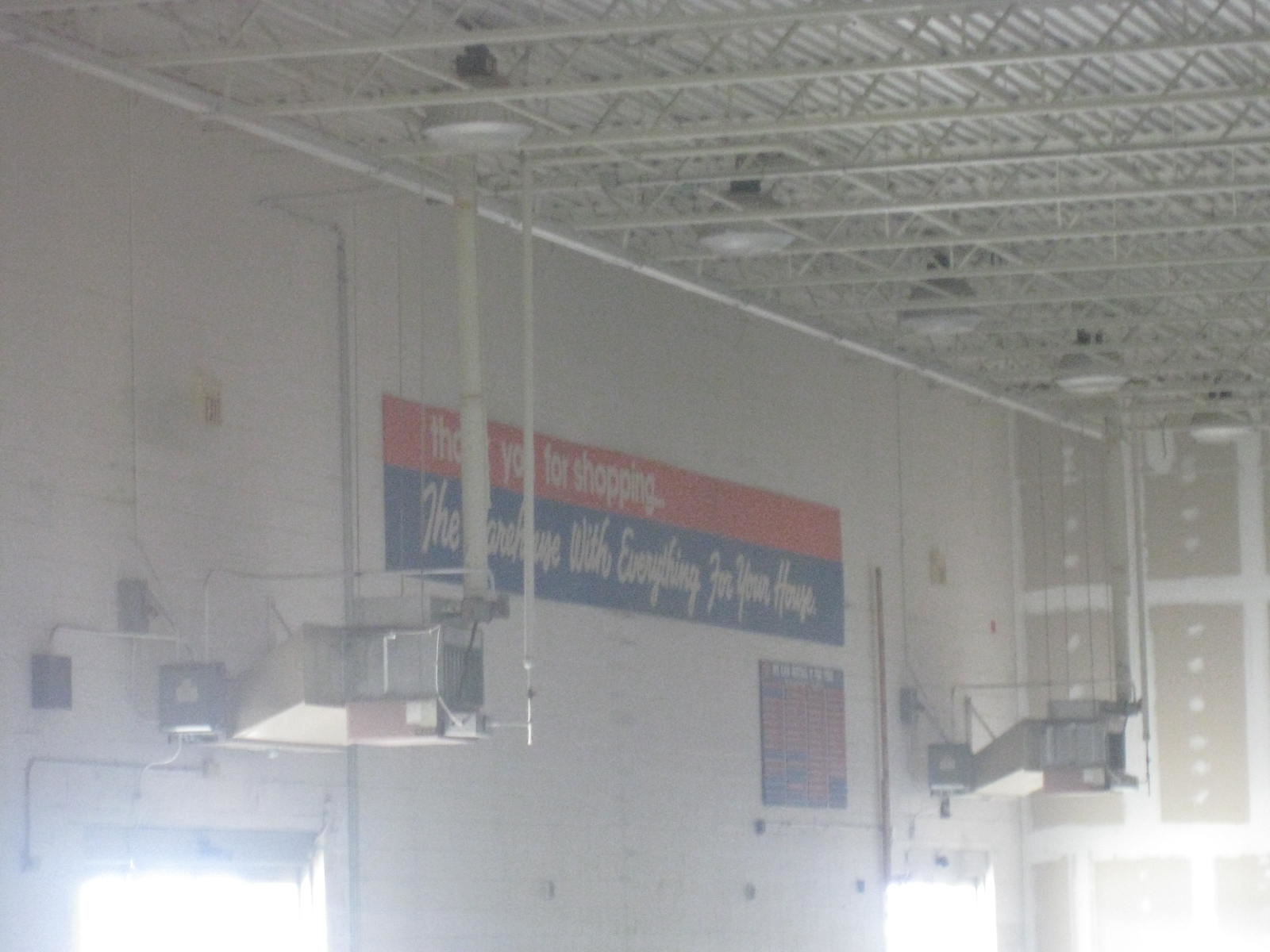This photograph captures the interior of what appears to be a large retail space, possibly an outlet or warehouse store. The image has a slightly blurred and washed-out quality, bathed in bright sunlight streaming through two doorways, lending the scene a faded, almost ethereal look. Dominating the left side of the frame is a white concrete wall adorned with a partially obscured sign that reads, "Thank you for shopping. The [something] with everything for your needs," possibly advertising a superstore. The sign is partially blocked by overhead ductwork, adding to the industrial feel of the space. 

Overhead, there are several descending lamps attached to beams, providing structured support for the ceiling. On the right side, a section of drywall stands out with visible mudding in a grid pattern, indicating recent installation work and suggesting that the store might still be under construction and not yet open to the public. The overall ambiance is a juxtaposition of raw, unfinished elements with the bright promise of a future retail haven.